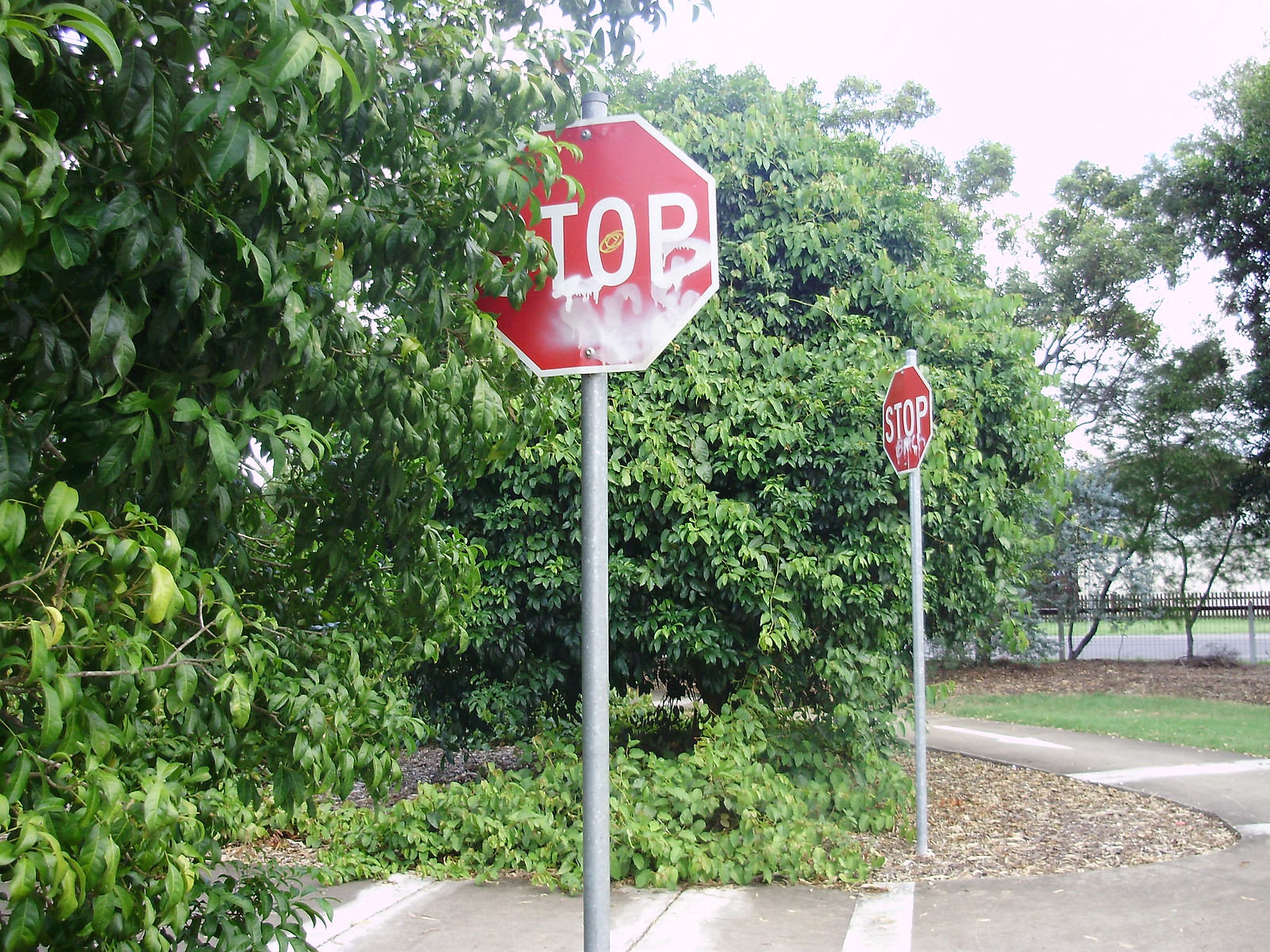This is a color photograph depicting two graffitied stop signs in a verdant park-like setting. Both signs are mounted on typical silver poles and exhibit the unmistakable red octagonal shape with capital white letters spelling "STOP." The first stop sign, positioned almost centrally in the image, has its "S" obscured by lush tree leaves, making it appear to read "TOP." This sign has white graffiti at its base, suggesting it might spell out "slob" instead. The second stop sign is further back and slightly angled to the left, also featuring white graffiti, though its letters remain unaltered. The scene is enriched with an abundance of greenery, including healthy trees and bushy vegetation. The green path or walkway that appears to be a curved sidewalk, runs between the two signs, with a black fence visible on the right side and possibly some vague buildings in the background. A patch of green grass and a paved area with white markings further define the landscape, all under a bright blue sky.